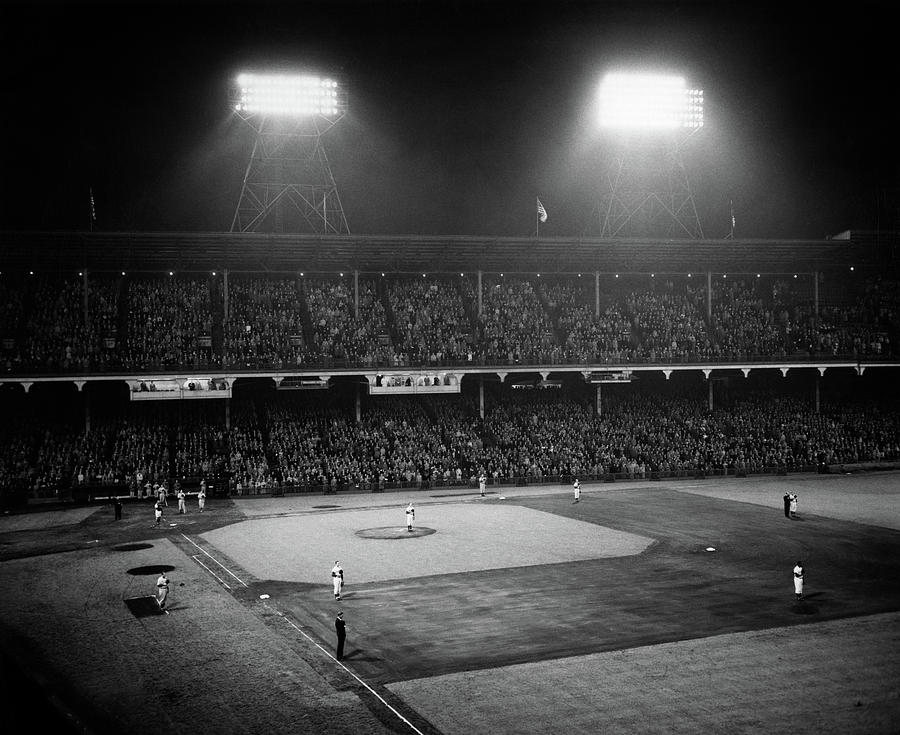The image is a black-and-white digital photograph capturing a distant, semi-aerial view of a nighttime baseball game. The scene is set within a fully packed stadium, showcasing two levels of bleachers—the lower and upper decks—both brimming with spectators whose individual details are too far away to distinguish. The sky above the stadium is pitch black, accentuated by two large stadium lights positioned above the upper bleachers, casting bright illumination onto the players below.

The baseball field is comprehensively visible from the home plate on the left to the farthest outfield, displaying all four bases. Players, donned in white and black uniforms, are scattered across the field, each standing solemnly with their hats off and pressed against their chests, all facing towards the right side of the image. The photograph encapsulates the solemnity of the moment while highlighting the stark contrasts and textures made poignant by the absence of color, rendering the entire scene in varying shades of black, white, and gray.